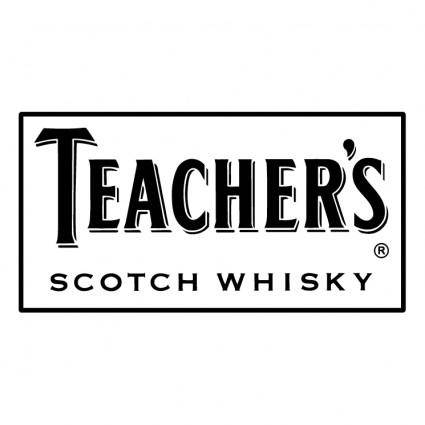The logo features a distinct label set against a solid white background. At the top, bold black letters spell out "TEACHER'S" with a capitalized "T" and an apostrophe between the "R" and "S". Beneath this, in smaller capitalized black letters, is the phrase "SCOTCH WHISKY," with a registered trademark symbol (an "R" inside a circle) placed between the "S" and "Y". Both lines of text are centered within a long rectangular shape, defined by a black border. The "TEACHER'S" text has subtle shadowing and white space within the letters, enhancing its outline. The overall design is monochromatic, solely using black and white.